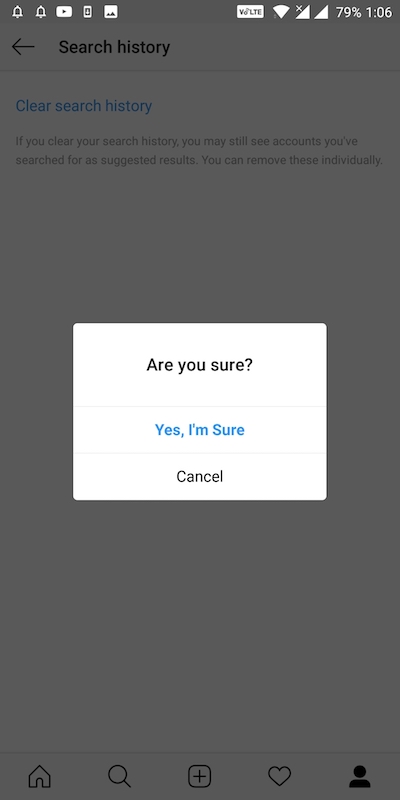The image depicts a smartphone screen displaying a search history clearing interface within an app. At the top of the screen, various status icons are present, including a battery icon at 79% and the time displayed as 1:06. Below these icons, a back arrow is visible, followed by the text "Search History."

Prominently positioned in the center is a blue button labeled "Clear Search History." A cautionary gray text below states, "If you clear your search history, you may still see accounts you searched for as suggested results. You can remove these individually."

A central pop-up box occupies the main part of the screen, featuring a white background with the question "Are you sure?" in black text. This pop-up includes two options: a blue "Yes, I'm sure" button and a black "Cancel" button.

At the bottom of the screen, a navigation bar contains five icons in black: a home icon, a magnifying glass indicating search, a square with a plus sign, a heart, and a silhouette of a person's head. The consistent color scheme and layout suggest the interface belongs to a social media or search-related app.